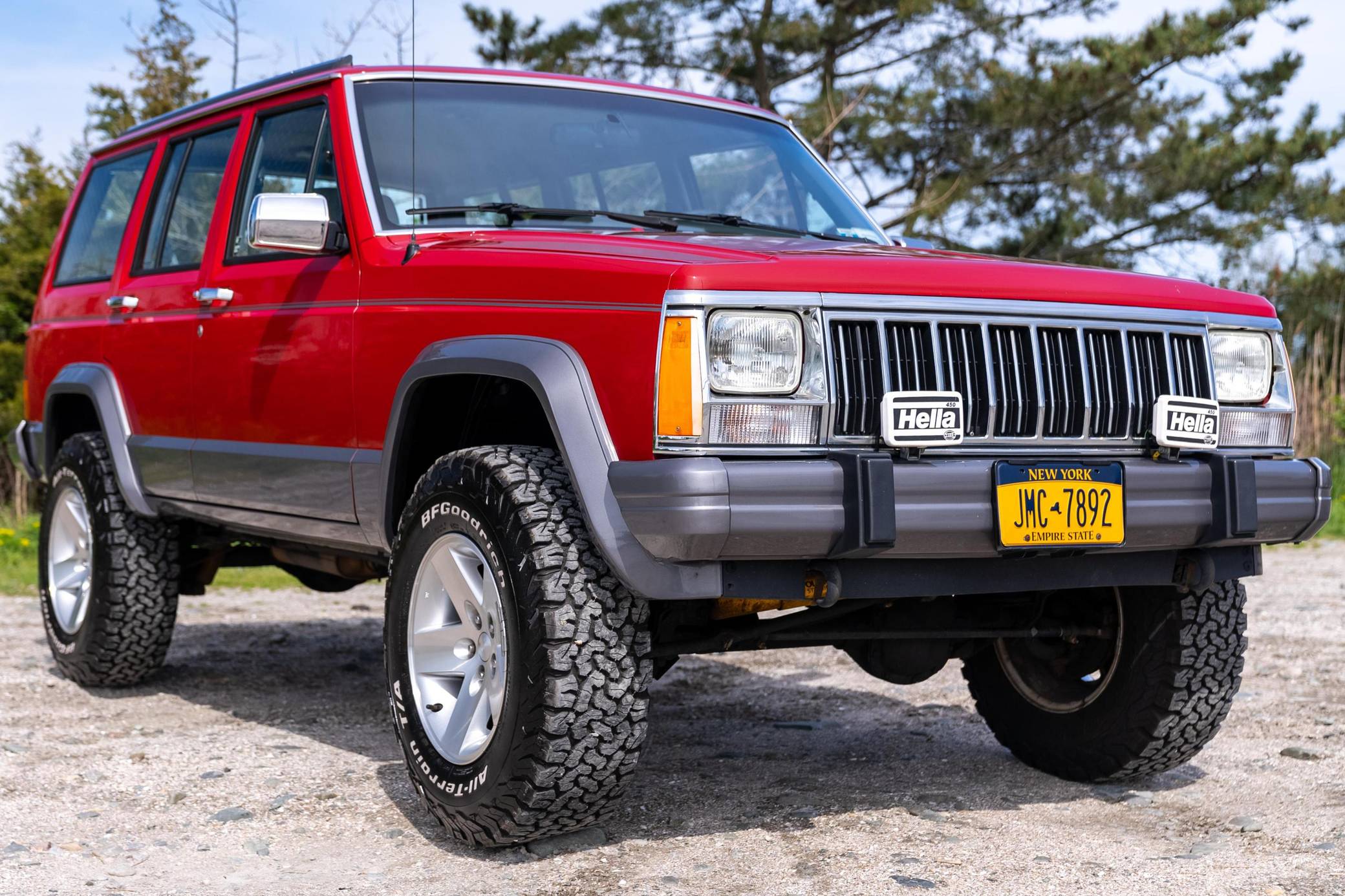This detailed photograph captures a vintage Jeep Cherokee from the early to mid-1980s, showcasing its distinctive red body with dark gray trim and silver alloy wheels. The Jeep is equipped with aggressive BF Goodrich all-terrain tires, marked with their recognizable white logo. The front of the vehicle features two prominently displayed Hella light covers. A New York license plate, characteristic of the era with its blue and yellow color scheme and inscription "JMC7892," is affixed to the front. The Jeep's iconic blocky design, emphasized by its lifted chassis and square grille, stands out in the image. The scene is set on a sandy surface, with a green field and trees in the background. The bright, midday sun casts hard shadows, suggesting the photo was taken around noon. The overall setting combines elements of a dirt or poorly maintained road, surrounded by nature, under a sunny yet slightly hazy sky.